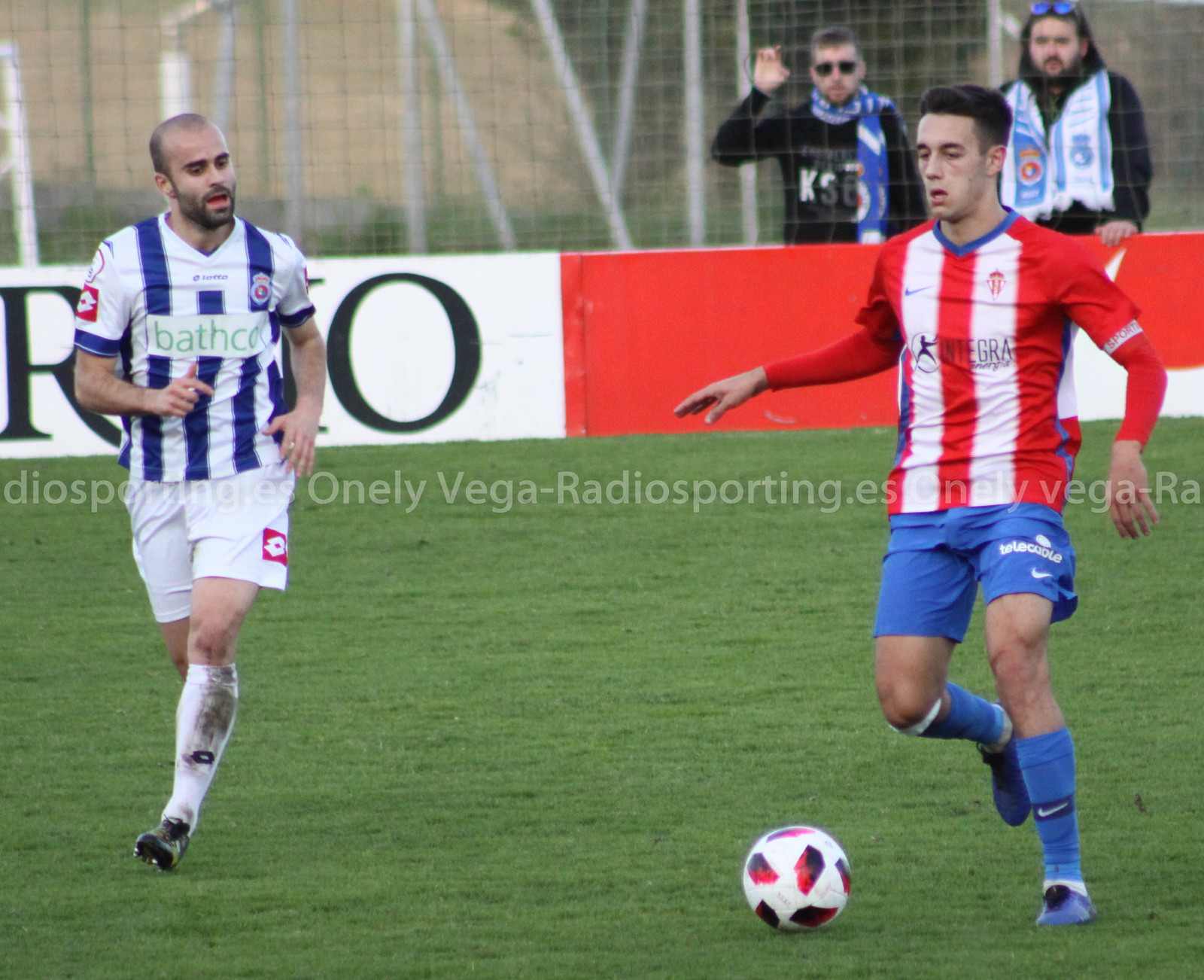The image shows two opposing soccer players on a green grass field, facing the camera. The player on the left wears a blue striped jersey with white shorts and dirty white socks. He has a shaved head, a close-cropped beard and mustache, and is Caucasian. The player on the right wears a red and white striped long-sleeve jersey, blue shorts, and light blue socks. He is also Caucasian, with short dark hair, and appears ready to kick the white, black, and red soccer ball positioned in front of him. In the background, beyond a thin metal fence and retaining wall, are two spectators in black jackets and scarves, likely supporting their team. The wall, which has a red and white design, partially displays text that includes the words "D-I-O-S-P," "O-N-E-L-Y," and "Vega, V-E-G-A," along with a partially obscured URL "radiosporing.es". The scene captures an intense, action-packed moment in the game.